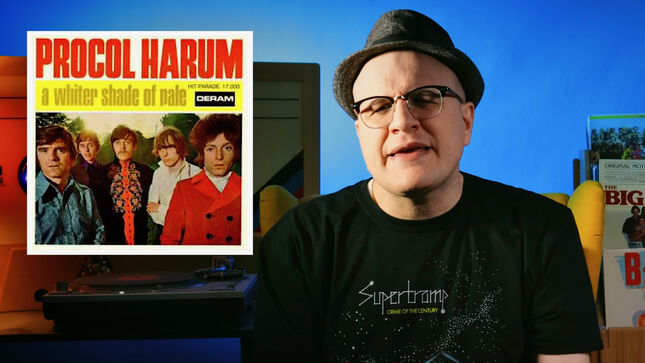The image is an indoor photograph, rectangular in shape, measuring approximately six inches wide and two to three inches high. The background at the top is blue. The photograph features an older Caucasian man from the chest up on the right side of the image. He is wearing a gray hat pushed back on his head, revealing that he might be bald, and black wire-framed glasses. His eyes are partially closed, and his mouth is slightly open, giving the impression that he is speaking. He has noticeable lines between his eyebrows and around his mouth. The man is dressed in a black short-sleeved t-shirt with white text that says "Super Tramp," followed by an unreadable line of yellow print underneath. 

In the background on the right, there are stacks of magazines or LP covers. To the left of the man, superimposed over the image, is a record player. Above it, there is a square section with a white background that reads "Procol Harum" in red text. Below that, against a yellow background with gray print, it reads "A Whiter Shade of Pale." Under these text elements is a photograph of five men dressed in 1960s fashion, appearing to have long-sleeved button-up shirts, with one of them possibly sporting an afro.